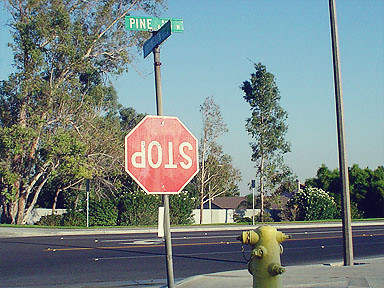In this slightly washed-out, retro-looking photo taken on a bright, sunny day, the sky is a flawless light blue with no clouds in sight. To the left and extending into the background are verdant deciduous trees, taller on the left and growing shorter towards the right. Dominating the mid-ground is a yellow ranch-style house situated beyond a four-lane road marked with a central yellow line and white lines dividing the lanes on the blacktop surface. In the foreground stands a vivid yellow fire hydrant beside a tall gray pole. However, the focal point of the image is an overturned stop sign, hanging from a gray pole. The sign, which is faded, still clearly displays the white lettering of "STOP," though it is now upside down due to a missing top bolt. Above the stop sign are two green street signs; the top one is clearly visible and reads "Pine," while the lower one is partially obscured and unreadable.